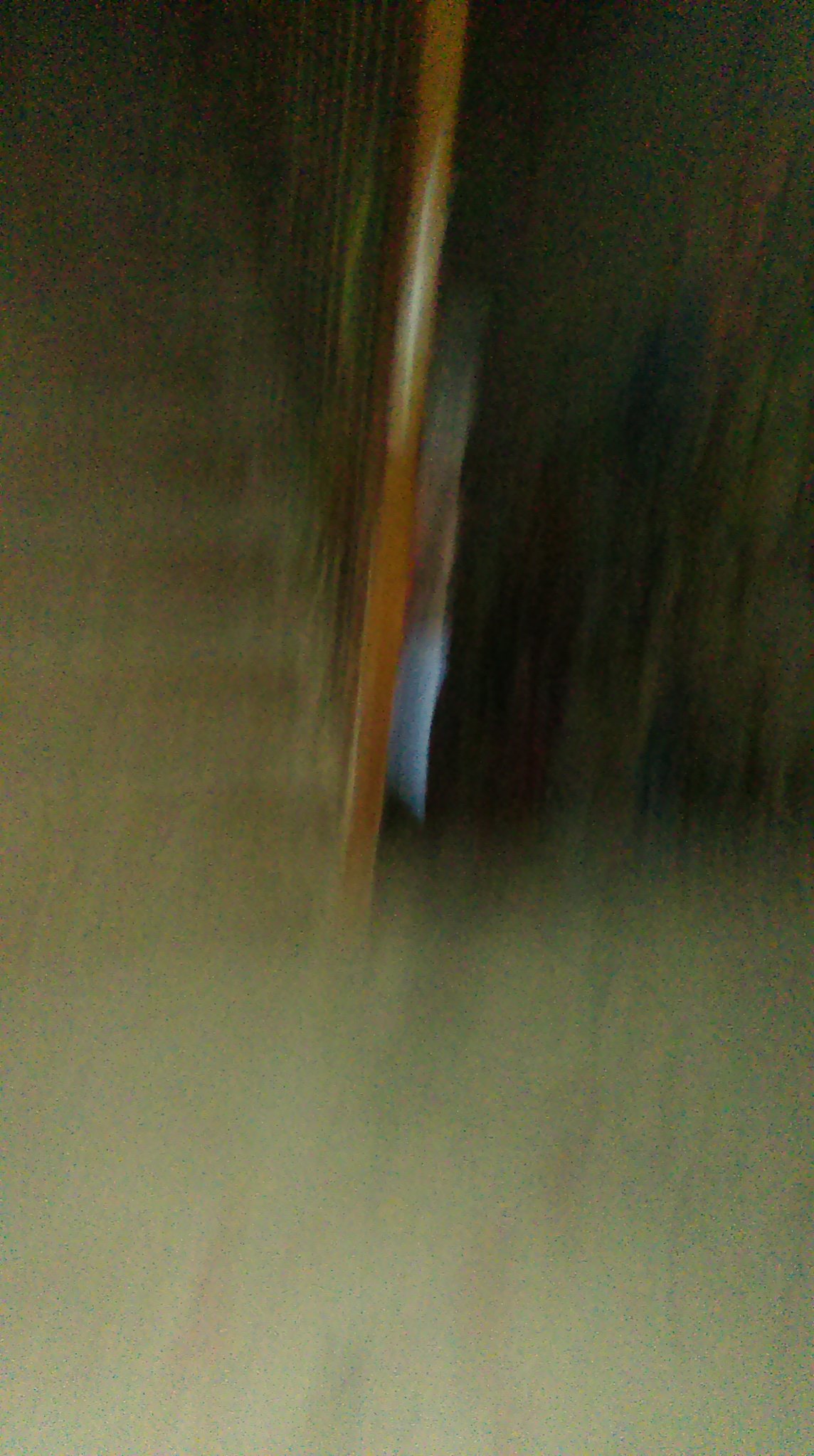This image is presented in a tall, vertical aspect ratio and suffers from significant motion blur, making the details indistinct. The photograph appears to have been taken in a dimly lit environment, likely causing the camera to struggle with stability, resulting in notable digital noise. The overall color palette is predominantly a dark, pale yellowish-green. A pronounced dark shadow occupies the right side of the frame, enhancing the murky atmosphere. At the center, there's a feature that resembles a wooden post. In the top left corner, faint shading suggests the presence of a staircase, which might explain the darker shadowed regions, indicative of a transition to a lower, less illuminated area.